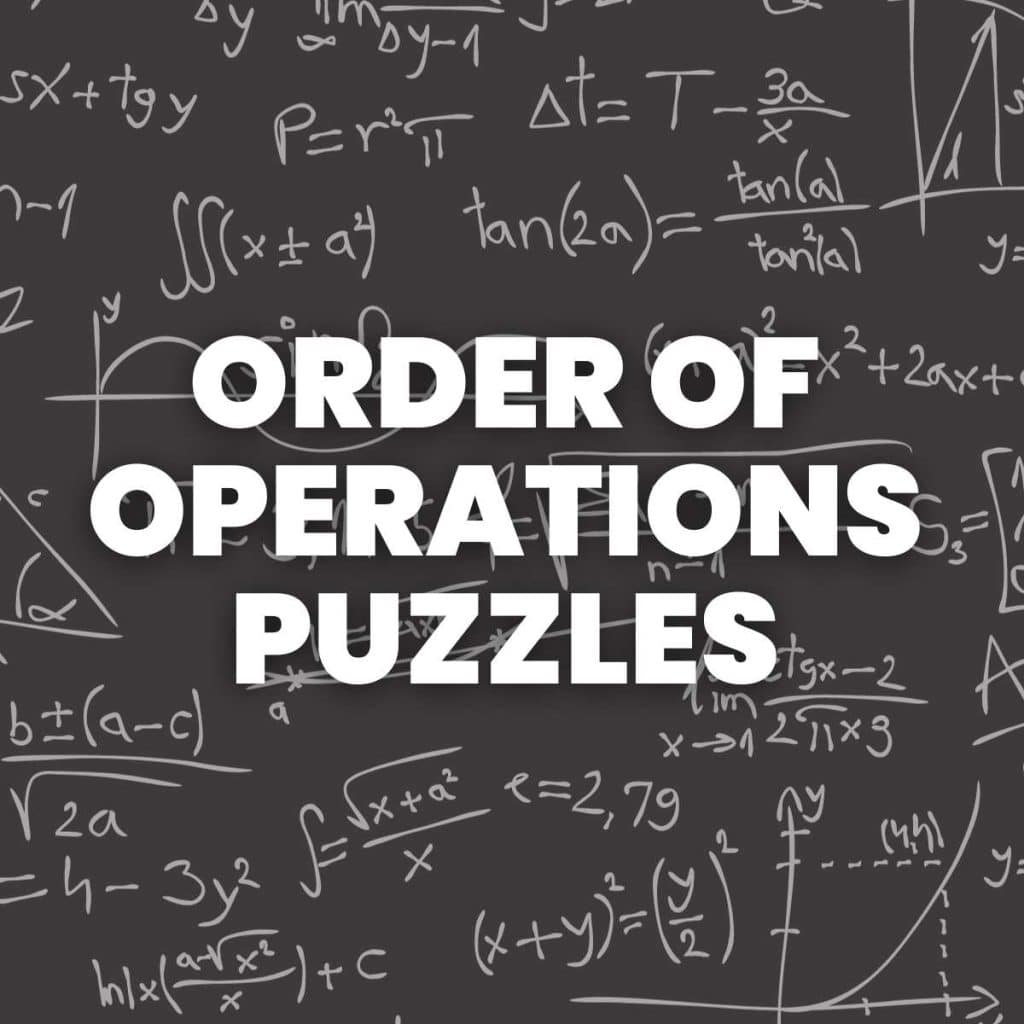The image displays a digitalized blackboard with a gray, chalkboard-like background, densely covered with various complex mathematical formulas and algebraic equations, including variables such as \( x \), \( y \), \( P \), and \( A \). Prominent equations include \( \text{tan}(2A) = \frac{\text{tan}(A)}{\text{tan}(2A)} \), \( P = R^2 \pi \), and integral expressions like \( \int (x \pm A^2) \). In the very center of the image, bold white text in capital letters spans across three lines, reading "ORDER OF OPERATIONS PUZZLES". The background equations create an intricate, detailed backdrop featuring additional elements such as double integral signs, an infinity symbol, and graphical representations, with specific formulas like \( SX + TGY \) and \( \Delta Y - P = R^2 \pi \).